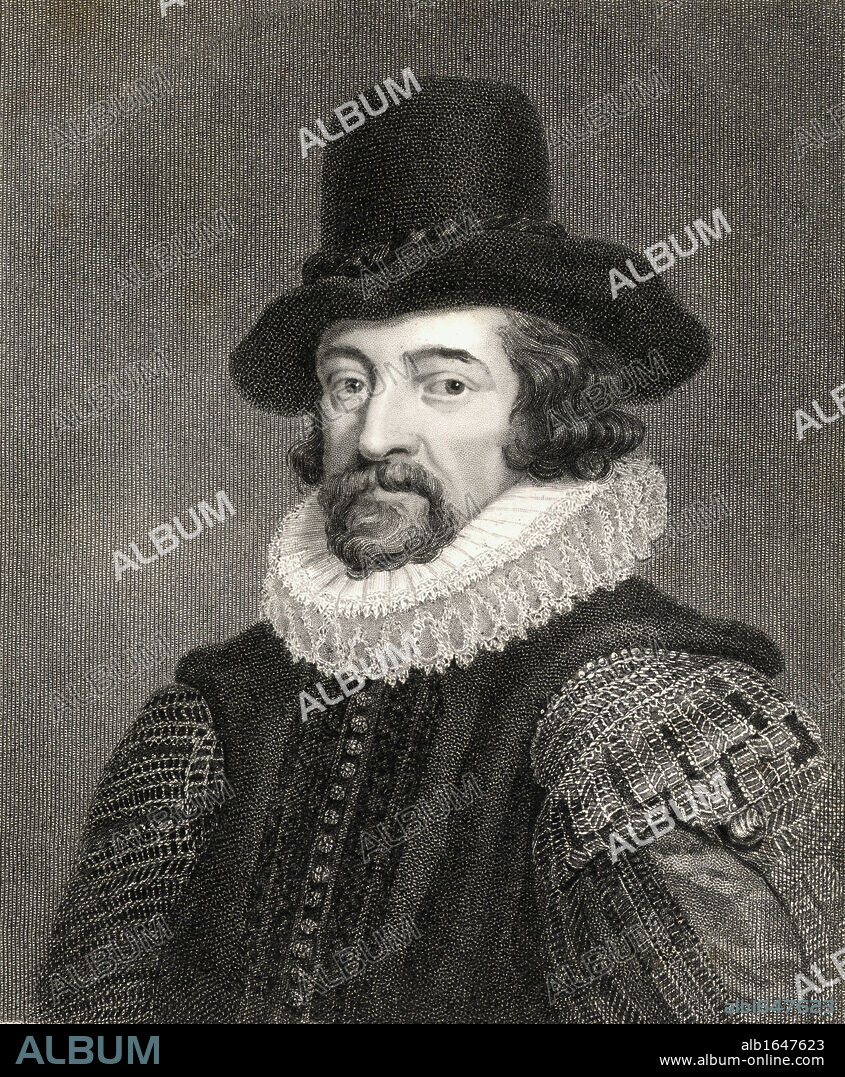This black and white image captures a man from the 16th century, donning a tall black top hat with a slightly irregular top. His longer, wavy brown hair cascades just below his ears, complementing his mustache and goatee. The man wears a distinct white frilly lace neckpiece, characteristic of regal attire of that era, and a frilly top jacket adorned with buttons and textured, voluminous puffed sleeves. The entire background is pixelated in monochrome, adding to the vintage aesthetic of the photograph. Various watermarks with the text "album" in white letters are scattered across the image to protect against unauthorized use. At the bottom right, the photograph is marked with "album" in a bluish tone alongside the text "ABI AB1647623" and the website "www.albumslashonline.com." The gentleman gazes directly at the camera with a neutral expression, enhancing the timeless essence captured in this photo.